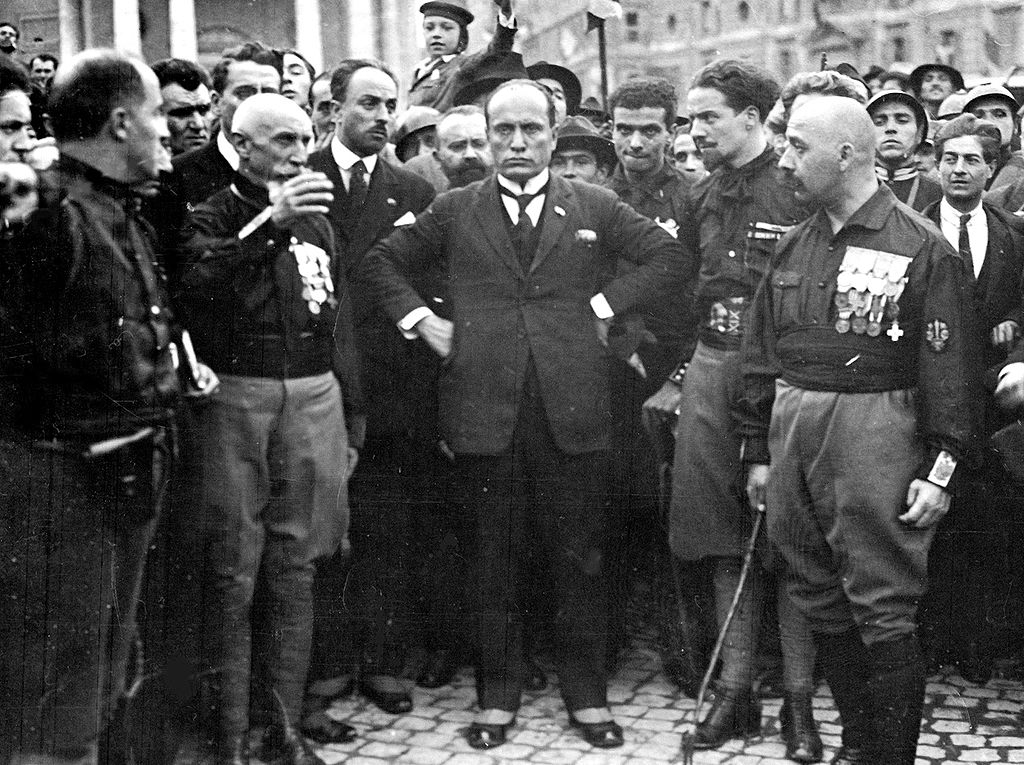The black-and-white image, likely from the early 20th century, depicts an outdoor scene on a cobblestone street, possibly in a city, with multi-story buildings visible in the background. At the center of the photograph stands a short, balding man with a high forehead, wearing a black suit with a white shirt and black tie. He has his arms extended at his hips in a serious stance, facing the camera. Flanking him are men in military uniforms adorned with war medals and badges, some holding sticks or whips. These soldiers appear attentive to the central figure, suggesting he is a leader or person of importance. A diverse crowd, including a child on someone's shoulders, mills about the scene, contributing to a sense of public gathering or event.